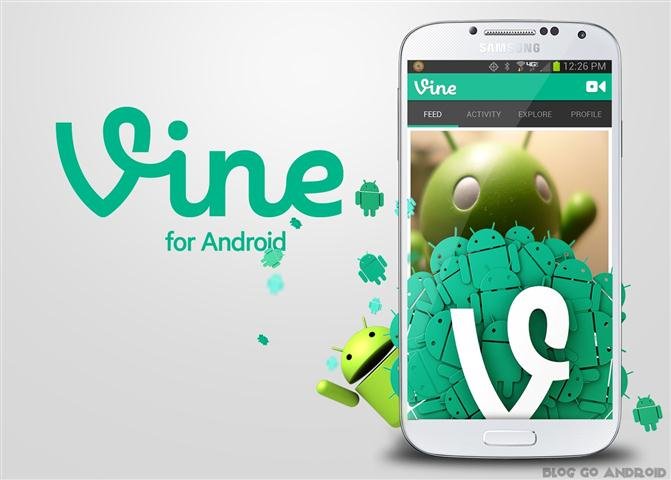The image showcases an advertisement for the now-defunct video blogging app, Vine, specifically for Android devices. Dominating the left side of the image is the word "Vine" written in cursive lettering over a mint green bar, with the text "For Android" positioned below it. To the right of this text is a white Samsung cell phone, which is an older model recognizable by its physical oblong button at the bottom and a silver headphone grill at the top. The time on the phone display reads 12:26 PM. The phone screen itself displays the Vine app interface with another "Vine" written in white at the center. The background features multiple stacked Android mascots, with one green Android mascot prominently waving from behind the phone, adding a playful touch. The primary colors of the image are white, green, and mint, creating a fresh and tech-savvy aesthetic.